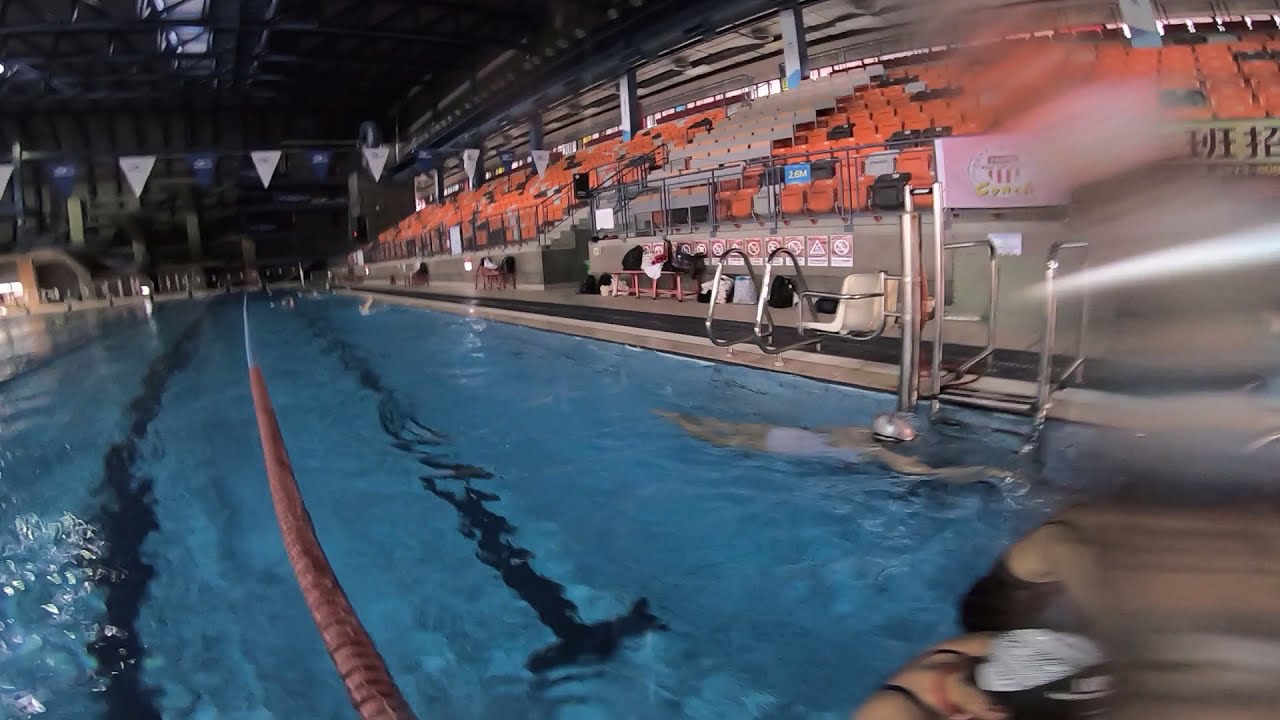The image captures an indoor swimming pool during what appears to be a swim practice session rather than a formal event, as there are no spectators present in the stands. The pool occupies the central and left portions of the image, featuring distinct black lane markings at the bottom and several silver handrails along the edges. Blue and white flags are suspended above the water.

To the bottom right, a female swimmer in a black swimsuit has reached the end of her lane, gripping the pool's edge. Close behind, another swimmer in a white swimsuit with a silver swim cap is still in motion, heading toward the pool's end. Additional swimmers are visible in the blurred background, suggesting ongoing activity, with at least three participants in the water.

The stands, located at the top and far side of the pool, display a mix of orange, black, gray, and red seating but remain empty. A walkway with benches, bags, and chairs separates the stands from the pool. The ceiling of the facility is detailed with reinforced steel rafters, contributing to the indoor setting. Overall, the image conveys a calm, practice-focused atmosphere amidst the functional design of the aquatic center.